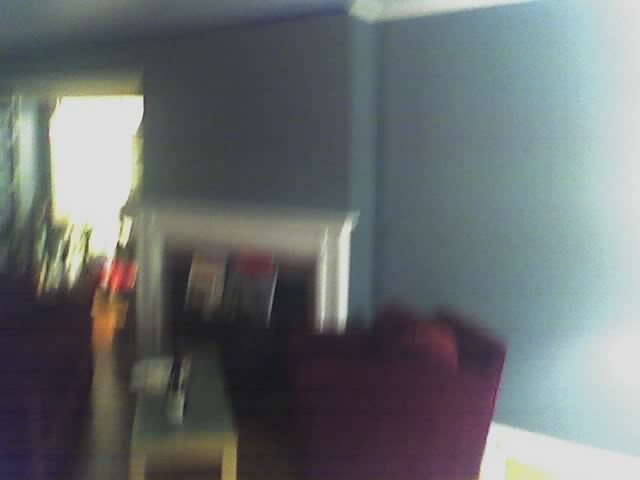A blurred photograph captures the interior of a cozy living room or reception area. The focal point is a light bluish-gray wall with a white mantle, housing a fireplace with indistinct objects in front. Dominating the foreground is a deep burgundy lounging chair, its back facing the camera, oriented towards the fireplace. Beside the chair, a coffee table displays a book or plate and a dark brown bottle of beer with a white label and the cap removed. Adjacent to the table is a matching burgundy couch. On the left side of the image, the space extends towards a large floor-to-ceiling window or possibly a sliding glass door adorned with curtains, although further furniture details are obscured.